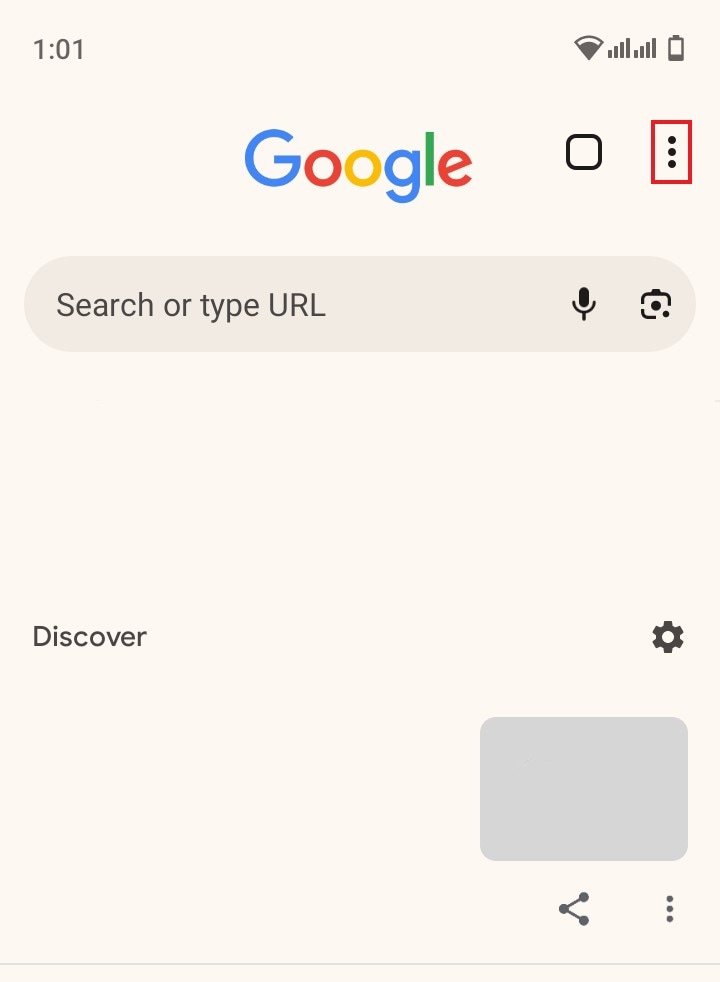The image features an orangey-tan background with several distinct elements. At the top left corner, the numbers "1:01" are displayed, followed by a Wi-Fi symbol. Adjacent to the Wi-Fi symbol, there are two sets of four diagonal lines that increase in length from left to right. Further to the right, there is an image of a battery.

Centered in the middle of the image is the Google logo, with its letters in various colors: blue, red, yellow, blue again, green, and red. Below the Google logo, there is a black square with rounded corners, containing a red rectangle with three vertically aligned dots.

Towards the bottom of the image, there is a slightly darker tan rectangle that expands outward on either side. Inside this rectangle, the text reads "Search or type URL" on the left side, and next to it on the right, there is an image of a microphone. Adjacent to the microphone icon is another symbol resembling a partial square with two circles (one inside and one outside) and a small notch at the top.

Below this section, the word "Discover" appears on the left side, while on the right side, there is an icon that resembles a gear shift. Further down, there is a gray rectangle with rounded corners, and beneath it, three vertically aligned gray dots are accompanied by the text "Share symbol."